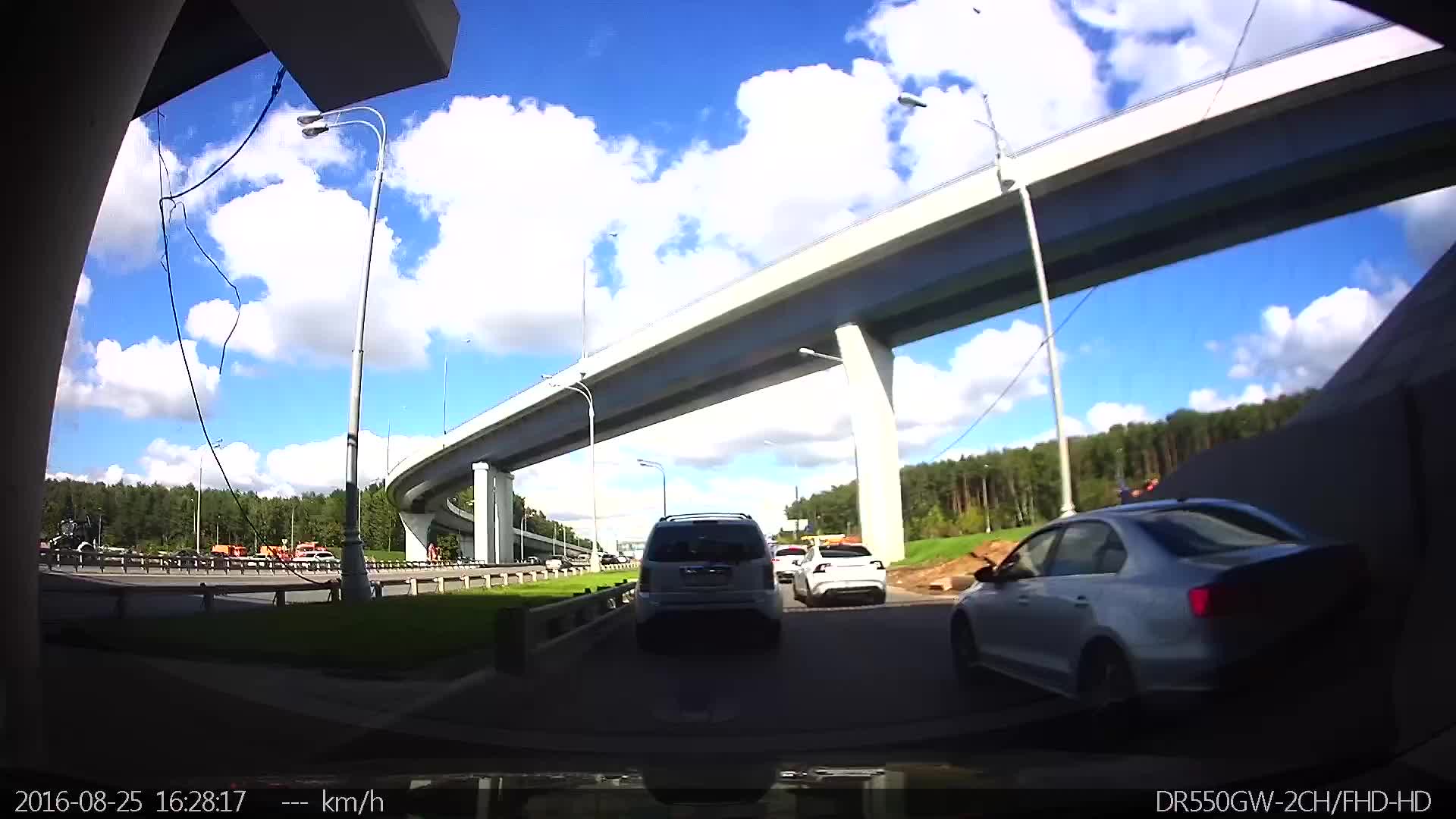The image, captured from inside a car possibly through the front windshield, shows a scene on a busy freeway characterized by a blue sky with white, puffy clouds. The highway has two lanes in each direction, separated by a grassy median with a low guardrail. Tall green trees line both sides of the road. Ahead, a towering concrete bridge, approximately 30 feet high, spans the view, supported by visible concrete beams. The bridge features white posts on either side. In the traffic-clogged lanes, several cars can be seen ahead, including those in the right lane. Two streetlights are positioned on the left and right sides of the road. At the very bottom of the image, there is a timestamp reading "2016-08-25 16:28:17," and the text "KM/H" indicating speed. Additionally, the bottom right corner features the text "DR550GW-2CH-FHD-HD."